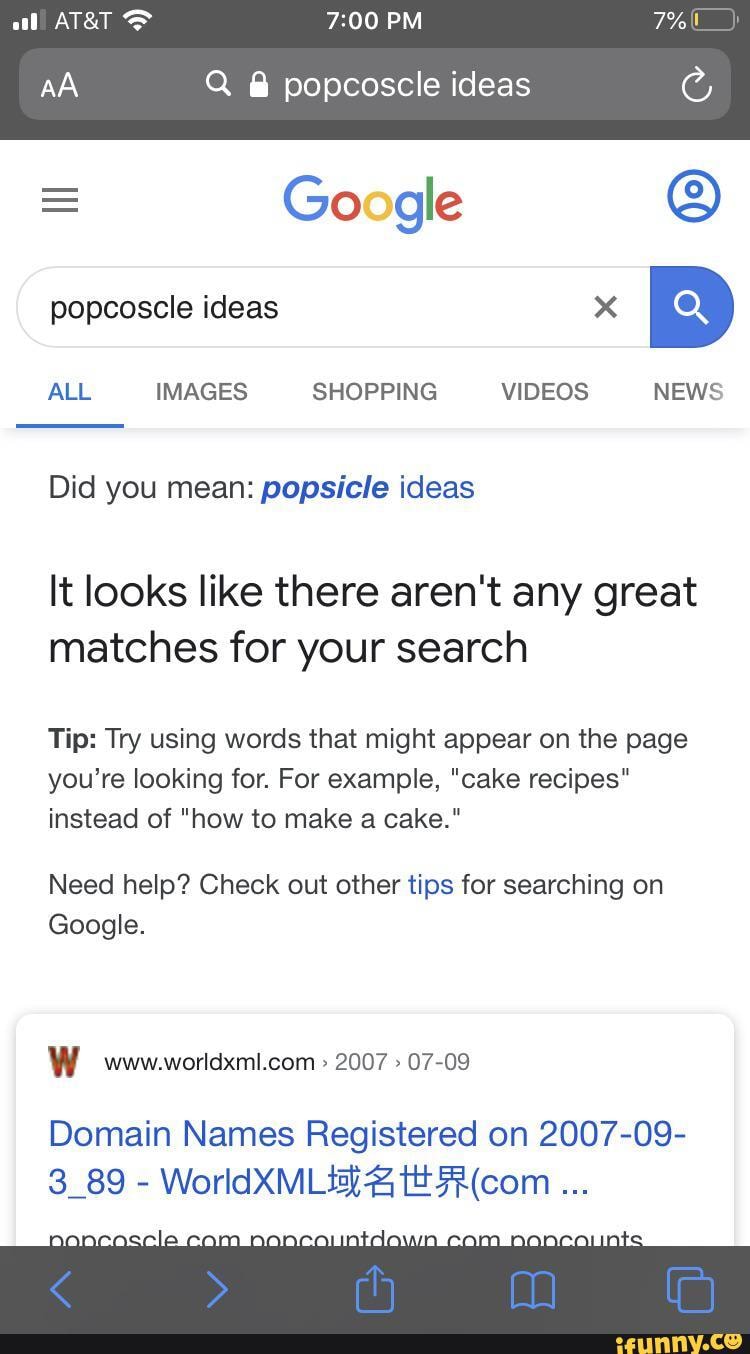This image is a vertically oriented screenshot of a Google search results page captured on a mobile device. At the top, the status bar reveals it is 7 p.m., with AT&T as the service provider, and the battery level is at 7%. The search input at the top shows a query for “pop coscle ideas,” which appears to be a misspelling of “popsicle ideas.”

Immediately below the search bar, the Google logo is prominently displayed, followed by the search query “pop coscle ideas” visible within the input box. The navigation menu options including “All,” “Images,” “Shopping,” “Videos,” and “News” are displayed. The "All" tab is currently selected and underlined in blue.

Google offers a correction, asking “Did you mean: popsicle ideas?” where “popsicle ideas” is highlighted in bold and underlined. Beneath this suggestion, Google indicates, “It looks like there aren't any great matches for your search,” and provides helpful tips for refining the search, such as using more relevant keywords.

Below these tips, there is one search result listed from www.worldxml.com, although the content of this result seems unrelated and consists mainly of technical information such as "domain names registered in 2007.09.3.89."

This detailed capture illustrates a typical search experience on Google, including elements that guide users towards more accurate search results.